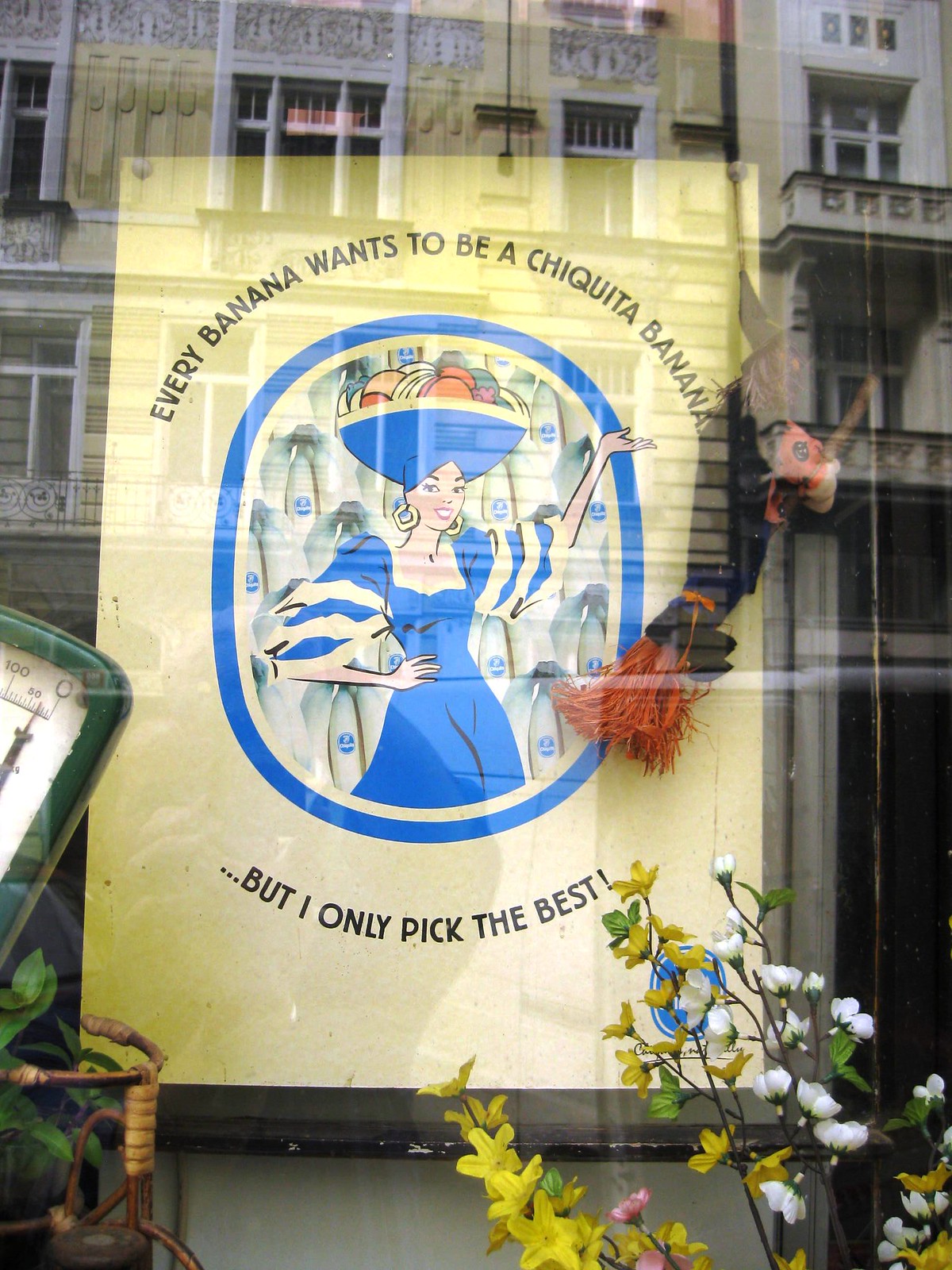The image depicts a shop window display featuring a vintage Chiquita banana advertisement. The poster shows the iconic Chiquita banana woman with a basket of colorful fruit on her head, large hoop earrings, and a blue dress with puffy sleeves. Above her is the slogan in black letters on a yellow background: "Every banana wants to be a Chiquita banana, but only I pick the best." The Chiquita logo is partially hidden by some flowers on the lower right side of the poster. Surrounding this poster is a Halloween-themed vintage witch decoration and an antique scale. Visible through the glass window is the reflection of a building with yellow and white hues and gray stone balconies, suggesting a picturesque, possibly European, cityscape. The shop seems to be an antique or collectible store, with additional details like brown wicker baskets, a clock, and other decorative items enhancing the nostalgic ambiance.